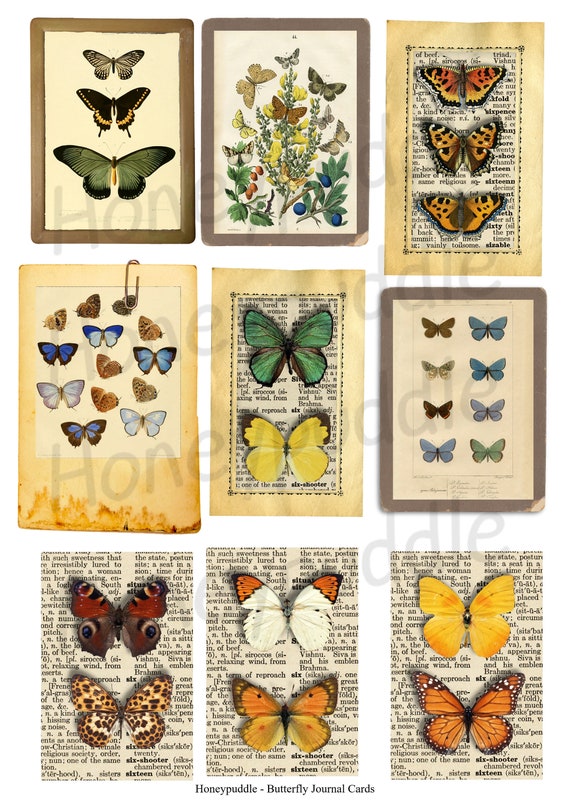The image features a vintage-style tableau of nine butterfly illustrations arranged in a slightly irregular grid pattern. Each horizontal row comprises three images, but some extend past the rectangular borders, adding an eclectic charm. The images collectively exude a translucent quality, set against a faintly marked background featuring repeatedly scribbled "Hone... D D L E" phrases in a diagonal, upward-right slant. The center bottom of the tableau is titled in a dark, possibly Times New Roman font that reads "Honey Puddle Dash Butterfly Journal Cards," with each word capitalized.

In detail:
1. **Top Left:** A smaller black and white butterfly, followed by a medium black and white butterfly. Both feature two lobed wings on either side, appearing squat as if horizontally aligned or slightly squished down. 
2. **Top Middle:** Featuring vibrant butterflies flying among red, yellow, and blue flowers, as well as what might be olives, all amidst green foliage.
3. **Top Right:** Set against a rectangle of newsprint with finely rendered vertical designs, this image shows three similarly sized yellow and orange-ish butterflies with black spots.
4. **Middle Left:** Exhibiting a tan background, this piece highlights a horizontally aligned rectangle showing blue and black butterflies, a blue and white butterfly, accompanied by brown, spiral-shaped cocoons.
5. **Middle Middle:** Similar in style to the top right, it displays a green butterfly on top and a yellow butterfly beneath it, both featuring distinct color patterns against a faint tan rectangle background.
6. **Middle Right:** Featuring two columns of butterflies in a structured yet varied display. The left column includes brown, white, then darker butterflies, while the right features blue to bluish-purple, and greenish-gray butterflies.
7. **Bottom Left:** Set on a newsprint background, this segment showcases a multicolored butterfly with peacock-like spots and an underneath butterfly with a leopard print pattern.
8. **Bottom Middle:** Against a background of an old yellowing paper, one butterfly near the top exhibits orange on its wings, while beneath it, a butterfly with orange and black details is followed by one in yellow with red dots.
9. **Bottom Right:** Features a yellow butterfly with subtle orange shading, and at the bottom, a monarch butterfly characterized by lacy black lines and white spots on its predominantly orange wings. The background is a contrast of black with white bubbles.

The overall effect is a rich collage, blending butterflies of varied colors and patterns with vintage aesthetics, echoing elements from the 1800s, enhanced by weathered textures and intricate background details.